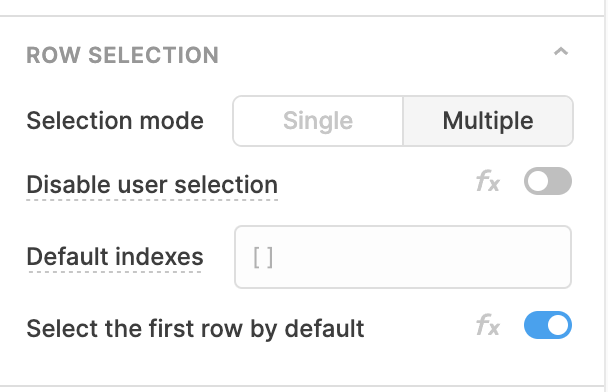The webpage appears to be an interactive interface designed for data manipulation and selection settings. The page is primarily gray and white, with various control options enclosed in a square box. 

At the top of this section, there is a heading in capital letters that reads "ROW SELECTION". Below this heading, there are options for "Selection Mode", with two choices: "Single" and "Multiple". The "Multiple" option is currently selected. 

Next, there is an option labeled "Disable User Selection" accompanied by a toggle button, which is currently in the 'off' (unselected) position. 

Following that, there is a section titled "Default Indexes" which contains a square input box with brackets, though it appears to be empty at the moment. 

The final option within this box is "Select the First Row by Default", marked with "Fx" and a toggle switch. This toggle switch is turned on, indicated by its blue color. 

At the top of the entire section, there is an arrow suggesting that more content may be accessible by scrolling up. 

Overall, the interface seems to be intended for managing data rows, possibly in a table or database format, allowing users to customize how data is selected and displayed.